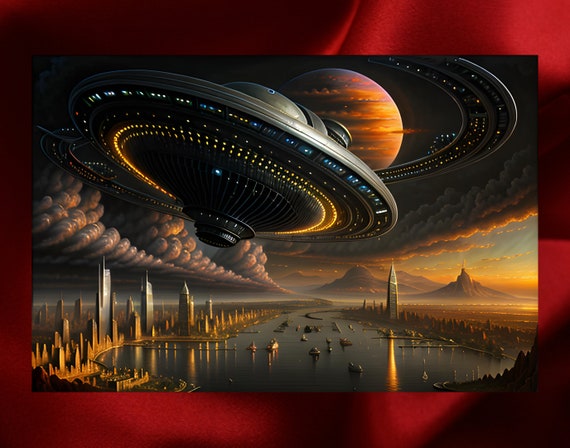The image is a detailed digital artwork with a rich, red, and dark background that creates a dramatic ambiance. Central to the image is a horizontal rectangle featuring a futuristic cityscape. Dominating the upper left portion of the scene is a large, saucer-shaped spaceship, dark gray in color and adorned with numerous lights and windows, giving it a distinct, otherworldly presence. The spaceship is angled slightly to the right, with black lines stretching from its top left side, curving upwards and then back to the left, dotted with white and yellow lights.

Above and to the right of the spaceship, a distant, orangish-colored planet adds to the cosmic feel of the composition. The sky further enhances this extraterrestrial setting with its deep, star-dotted expanse and the presence of a large planet with rings, resembling Jupiter but with a reddish-purple hue.

Below the spaceship, the city is bisected by a wide river, reflecting the lights from numerous watercraft and the surrounding buildings. Skyscrapers and medium-sized structures line the banks of the river, creating a bustling metropolitan skyline. In the distance, small mountains frame the horizon.

To the left side of the image, beneath the spaceship, clusters of whimsical, cylindrical white clouds roll across the sky, adding a surreal touch. The clouds appear stacked in groups, separated by gaps, and contribute to the scene’s layered depth. Throughout, the texture of the red background varies, giving an impression of folds and enhancing the image's dynamic quality.